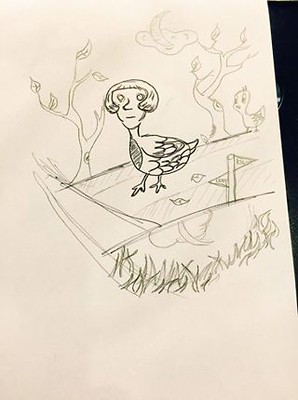The drawing on the piece of off-white printer paper depicts a whimsical scene rendered in pencil, possibly with some pen. The focal point is a fantastical bird with a duck's body and a woman's head sporting a short bob haircut. This hybrid figure walks on a sidewalk with webbed feet. Its human-like face is characterized by round, pupil-less eyes, a straight mouth, and a distinctive hook nose.

In the background, two spindly trees with sparse clusters of leaves frame the scene. A crescent moon emerges from a cloud in the sky, which is also reflected in a puddle of water on the side of the road. The road features a short street sign with unreadable text facing opposite directions and is marked by two bars that could suggest a finish line.

A smaller, more traditionally duck-like figure, reminiscent of Tweety Bird, stands to the side under a tree. Grass grows alongside the sidewalk, and leaves are scattered on the path behind the duck-woman. The overall image captures a playful and imaginative blend of human and animal features set in a serene, lightly detailed landscape.